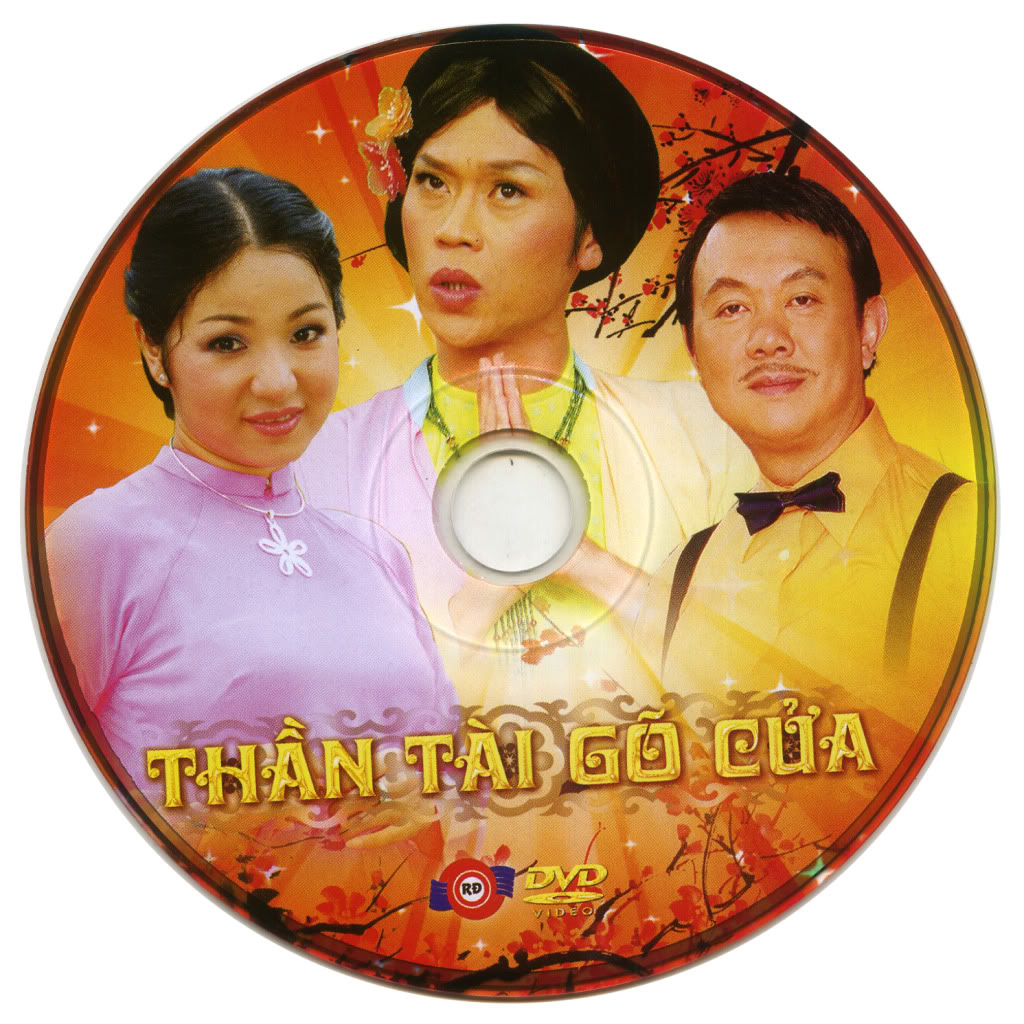The DVD cover features a prominently printed image and the title "Thanh Thai Go Qua" in embossed gold Vietnamese text. It showcases three people in the foreground against a decorative backdrop filled with cherry blossoms. On the left is an Asian woman with black hair pulled back, wearing a traditional pink dress with a little flower necklace, and pink lipstick and makeup. In the middle is another woman with a perplexed or annoyed expression, hands pressed together as if praying or greeting, adorned with flowers in her hair. To the right stands a man with a pencil mustache, sporting a yellow shirt, overalls, and a black bow tie. The entire design of the DVD is colorful with shades of orange, red, and yellow, evoking the warmth of a sunset, accented by intricate floral and branch patterns. The DVD also features logos such as "RD" and "DVD Video."